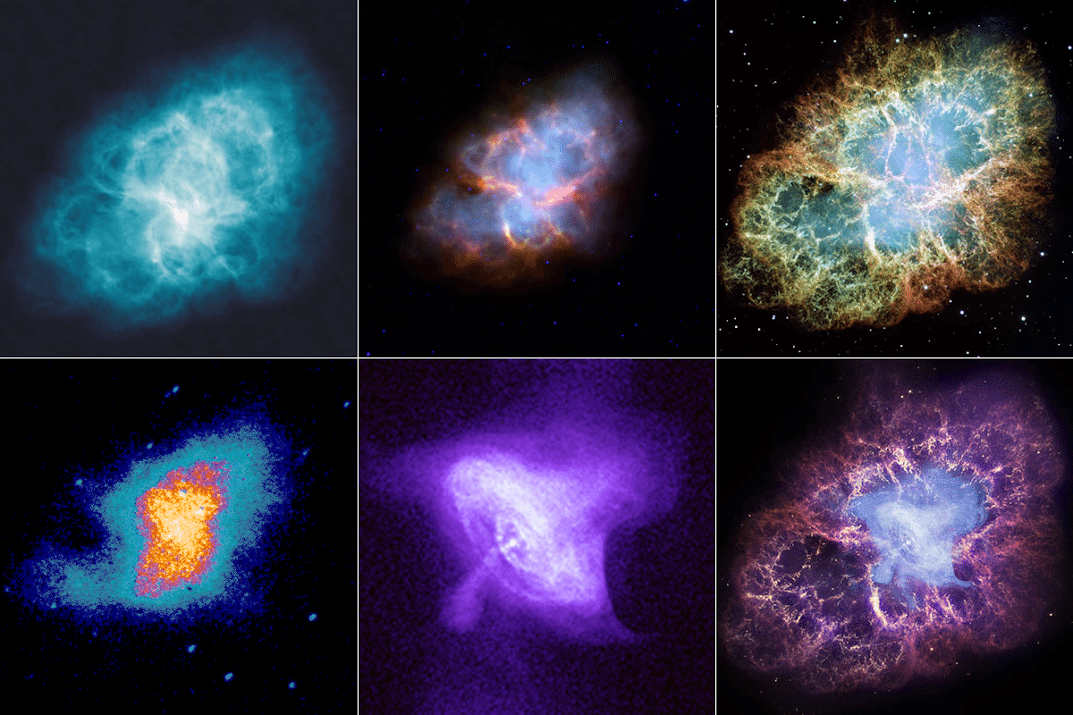This is a photo showcasing six different cosmic images that appear to depict various celestial phenomena such as galaxies or nebulae, arranged in a neat, two-by-three grid (three columns and two rows). The background of each image is a deep midnight blue, resembling space, with scattered stars visible in some of the images.

- **Top Left**: Shows a striking neon turquoise mass with a bright white center.
- **Top Middle**: Features a dark midnight blue backdrop with an oval shape glowing in a mix of blues and reds.
- **Top Right**: Displays an emerald green mass with shades of bronzish yellow and a smoky interior.
- **Bottom Left**: Contains a gradient transitioning from a dark blue to a vibrant orangey-red center, reminiscent of fire.
- **Bottom Middle**: Depicts a ghostly purple blob with a lighter white center.
- **Bottom Right**: Consists of a light blue core surrounded by a purplish red border, again against the midnight blue background.

Each image showcases unique, vivid colors and shapes, painting a detailed and vivid cosmic landscape, likely captured through advanced telescopic photography.